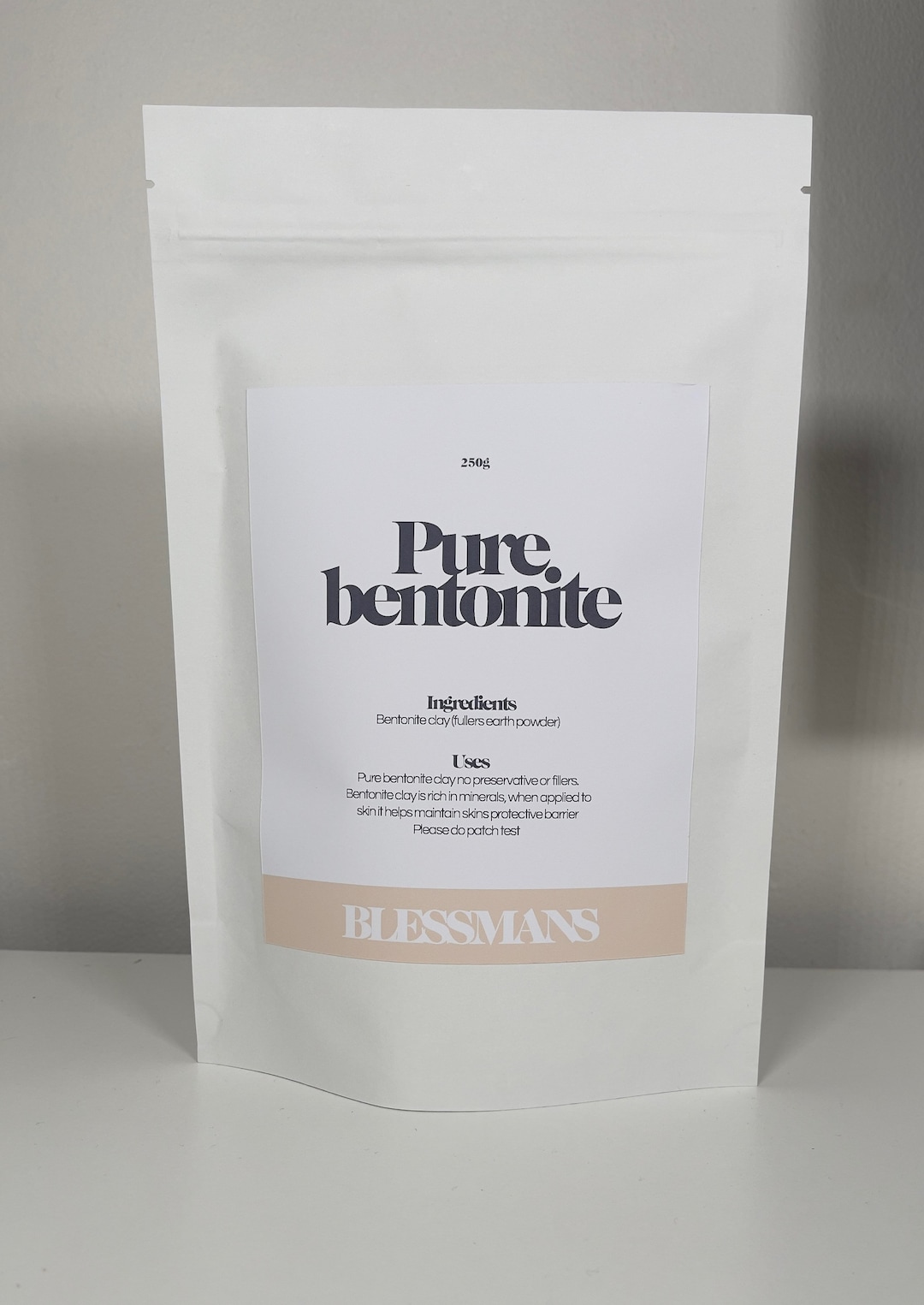This photograph captures a small, minimalist bag of bentonite clay, prominently displayed on a white surface against a blurry white background. The modern, white package features a clear, bold label in dark black letters that reads "250 grams Pure Bentonite." Beneath this, the list of ingredients includes "Bentonite Clay" and mentions earth powder for color. Further down, the uses of the clay are outlined, highlighting its richness in minerals and its role in creating a protective barrier for the skin, with an advisory to perform a patch test. At the label's bottom, the brand name "Blassman's" is displayed in a light brown peachy (or salmon) color, adding a subtle splash of color to the otherwise plain packaging. The label and the text are straightforward and functional, ensuring the focus remains on the product itself.